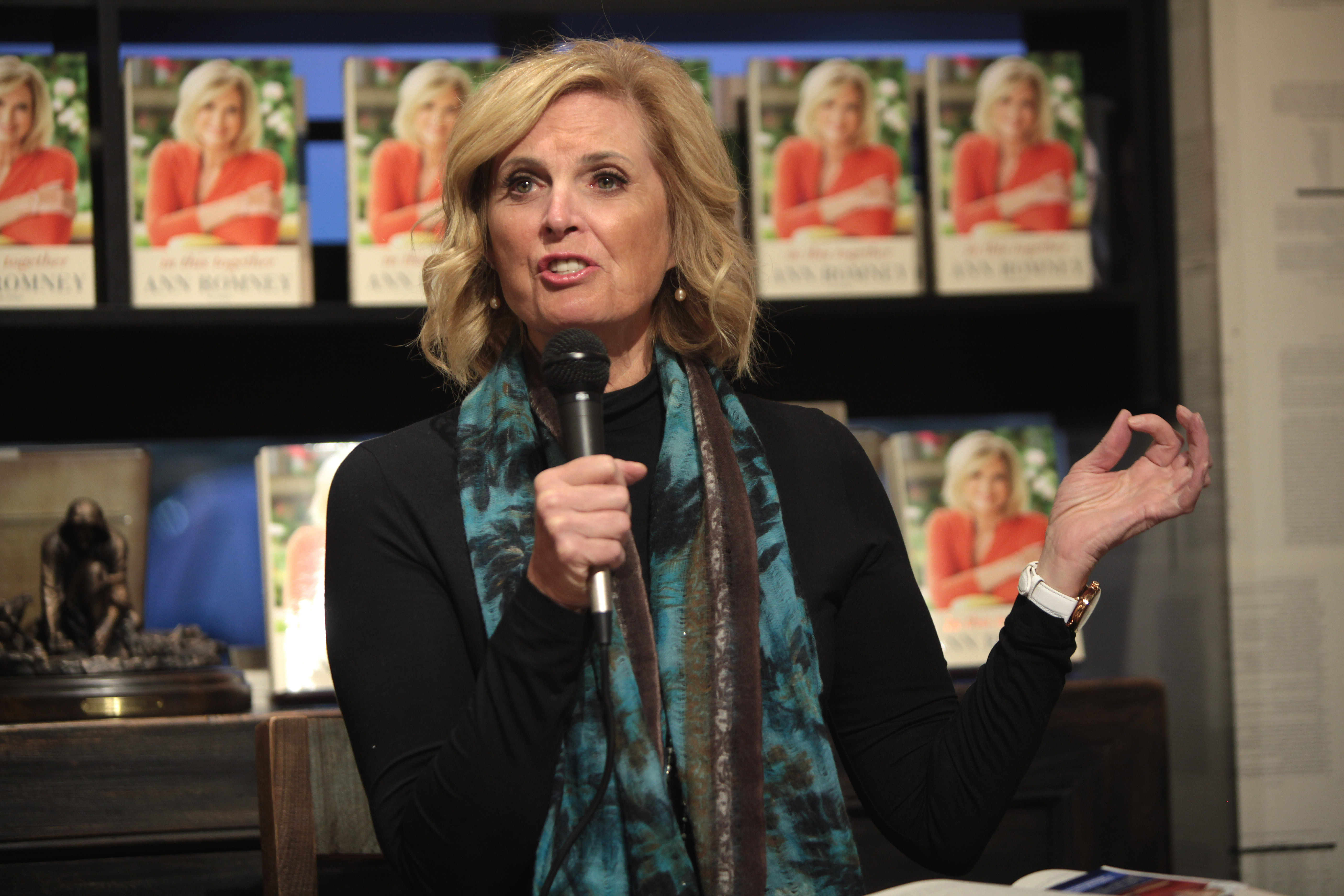This image captures a mid-sentence moment of a woman, likely in her late 40s or 50s, speaking into a black microphone with a silver bottom, during what seems to be a book tour or author event. The woman, identified as Anne Romney, has shoulder-length blonde hair and is dressed in a long-sleeved black top with a distinctive scarf featuring light blue and black floral patterns. She is accessorized with a wristwatch with a white band on her left wrist and pearl-like earrings. Anne is seated in a gray and wooden chair, and the setting appears to be indoors with a backdrop of bookshelves filled with multiple copies of her book. The cover of the books shows her in an orangish-red long sleeve top with a green grassy background and white flowers. To her right (the viewer's left), there's a small brown statue with a gold band. The scene exudes a formal, yet approachable atmosphere as she gestures expressively with her free hand.